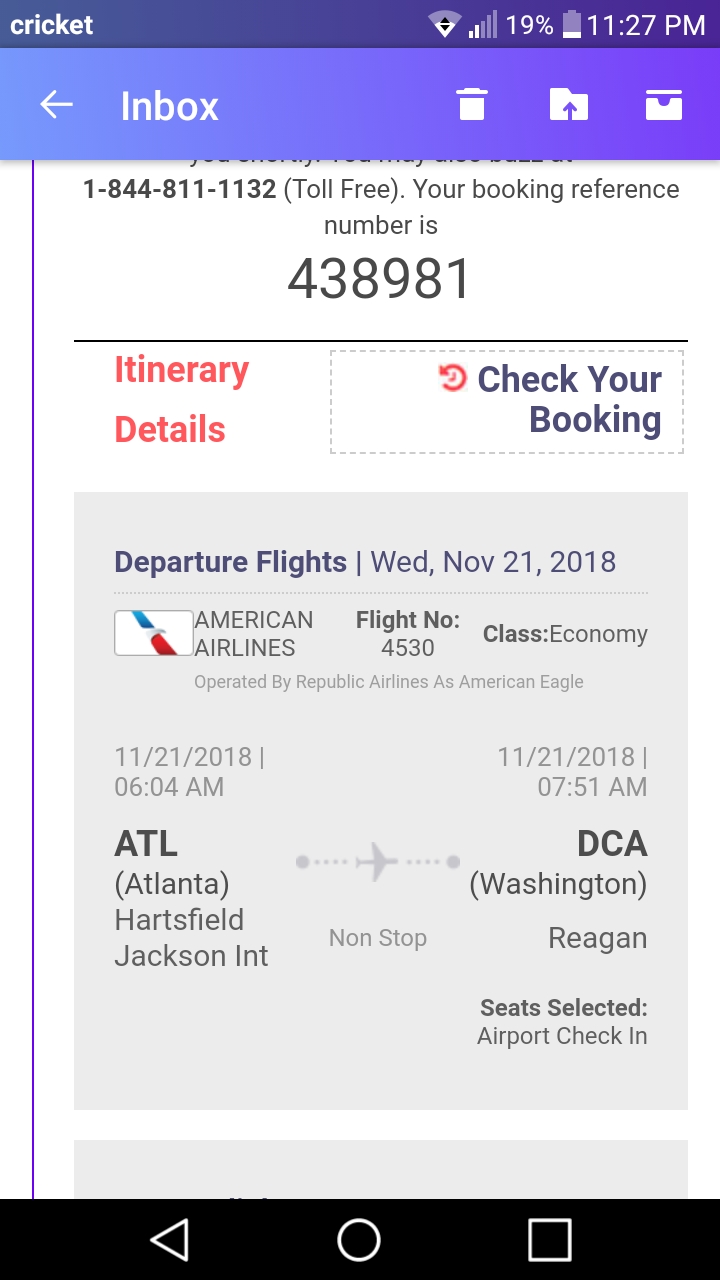**Detailed Caption:**

A screenshot of a cell phone taken at 11:27 p.m. shows the battery at 19%, with a cell signal strength of 2 out of 5 bars and a Wi-Fi signal of 2 out of 4 bars. The carrier displayed in the upper left corner is Cricket. Below that, there's a left-facing arrow indicating the back button, followed by the label "Inbox". Next to it, there's a trash can icon for deleting. Further to the right, there's an arrow pointing up into a folder icon, and a standard folder icon.

Beneath these icons, the screen shows a toll-free black phone number: 844-811-1132. Below this number is a booking reference number: 438981, followed by the text "Itinerary Details" in red letters and "Check Your Booking" in blue letters inside a blue rectangle.

In a larger gray rectangle below, the details of a departure flight are displayed: 

- **Date:** Wednesday, November 21st, 2018
- **Airline:** American Airlines
- **Flight Number:** 4530
- **Class:** Economy Class
- **Operated By:** Republic Airlines as American Eagle
- **Departure Time and Place:** 6:04 a.m. from Atlanta Hartsfield-Jackson Airport (ATL)
- **Arrival Time and Place:** 7:51 a.m. at Washington Reagan Airport (DCA)

There is text indicating that an airport check-in and seat selection have been processed.